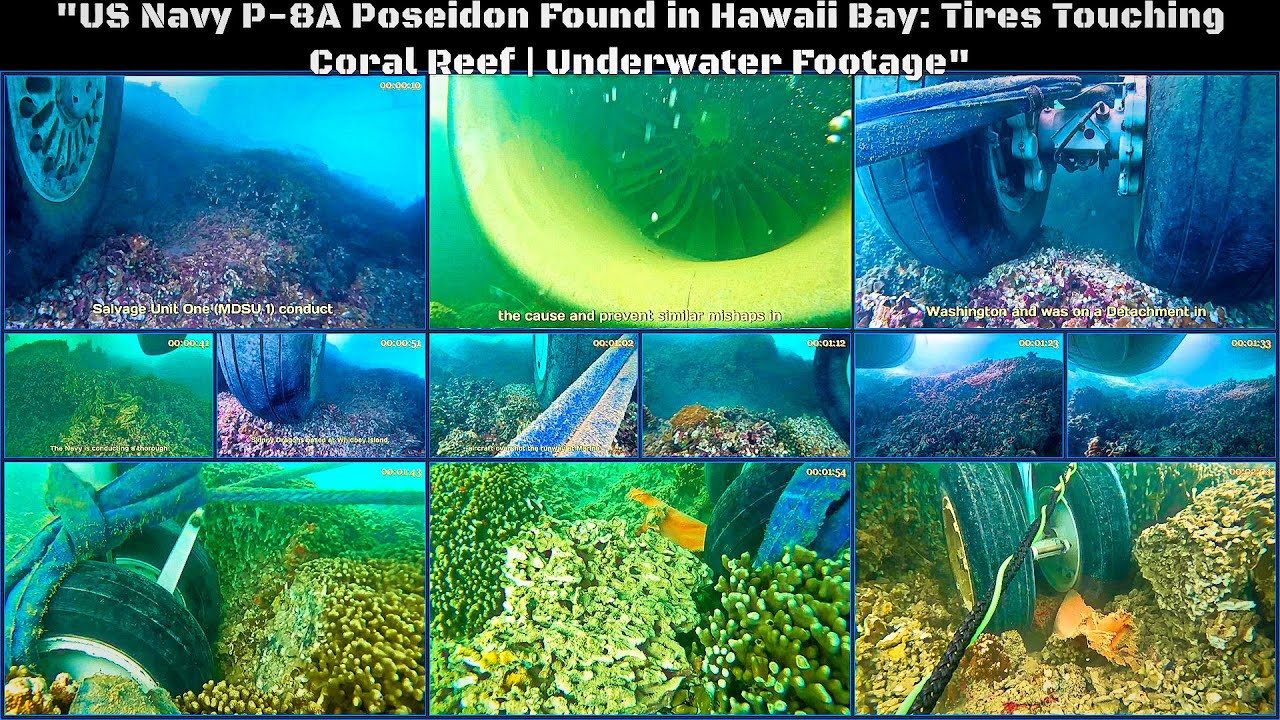This detailed collage of underwater photographs captures the aftermath of a US Navy P-8A Poseidon aircraft found in Hawaii Bay, showing various angles of black and silver tires tangled with vibrant green coral reefs. The image is topped with a black banner displaying the caption: "US Navy P-8A Poseidon found in Hawaii Bay: tires touching coral reef underwater footage." The photos expose close-ups of the jet's wheels resting on the coral, revealing the stark contrast between the mechanical debris and the natural underwater habitat. Additionally, there are images detailing the aircraft's engine and landing gear amidst the coral. Subtitles and annotations at the bottom of some images provide context, such as, "Salvage Unit 1, MDSU-1 conduct," and reference mishaps and efforts to prevent similar incidents. Numbered timestamps are visible on each photograph, illustrating the sequence and timing of the underwater investigation.